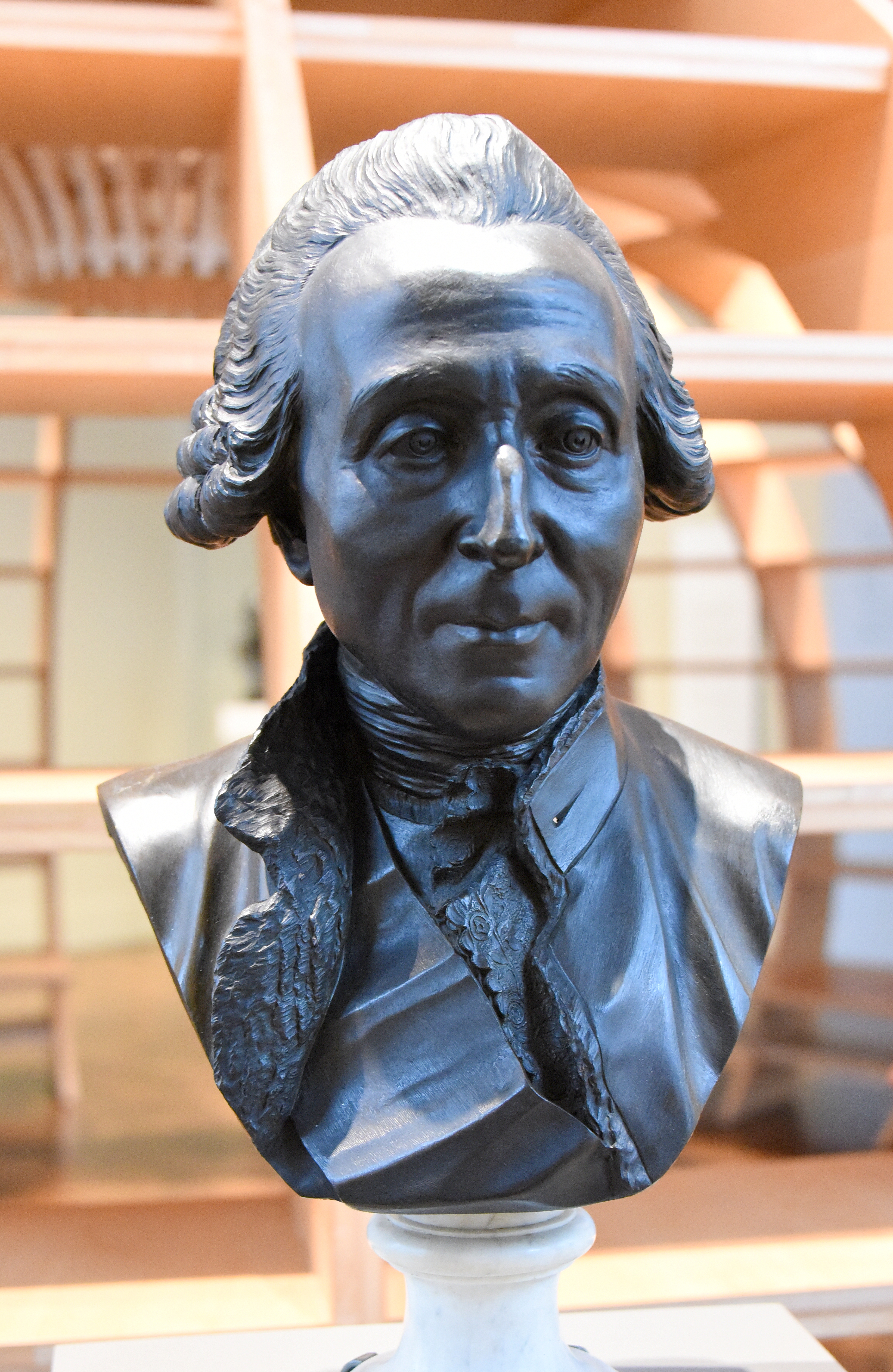The image features a hyper-realistic, highly detailed bust of a prominent historical figure, possibly a politician or founding father from the colonial era. The shiny black statue is made of either black marble or black bronze, and rests on a white circular pedestal, which in turn is set upon a rectangular brown stand or shelf. The figure has short, curly hair near the ears, and wears a jacket with a stand-up, high collar over a vest adorned with lace texture and folds. His facial features include a chiseled nose and a small, closed mouth. The surrounding background showcases what appears to be an architectural interior, possibly the entrance to a museum or library, characterized by brown arches and shelves, with a hint of additional artworks and structures. The overall ambiance of the setting is enhanced by the light illuminating the bust, bringing out its metallic gray sheen and making it look intensely lifelike.